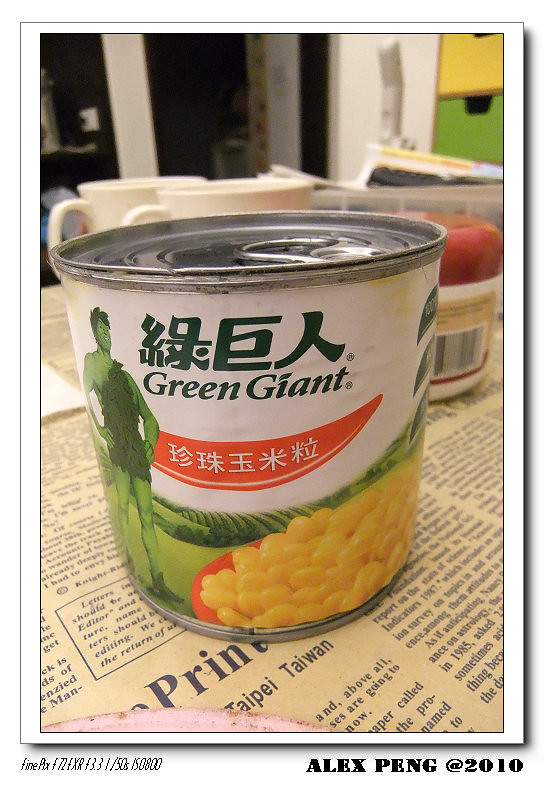A close-up photograph captures a small can of Green Giant corn resting on a yellowed English newspaper at a dining table, which appears to be part of a kitchen or office space, as suggested by background items including plain white coffee mugs, a shelf, and a sliding door. The can prominently features a Green Giant logo and imagery, with text in Chinese characters indicating its international origin. The can's label is divided with an upper white section and a lower green section; it also includes an image of a bowl of corn. The newspaper which the can sits on, has visible text reading "Printed in Taipei, Taiwan." The image has a white border, with "find pics" and some numbers in the bottom left corner, and "Alex PENG at 2010" in black letters on the bottom right corner.